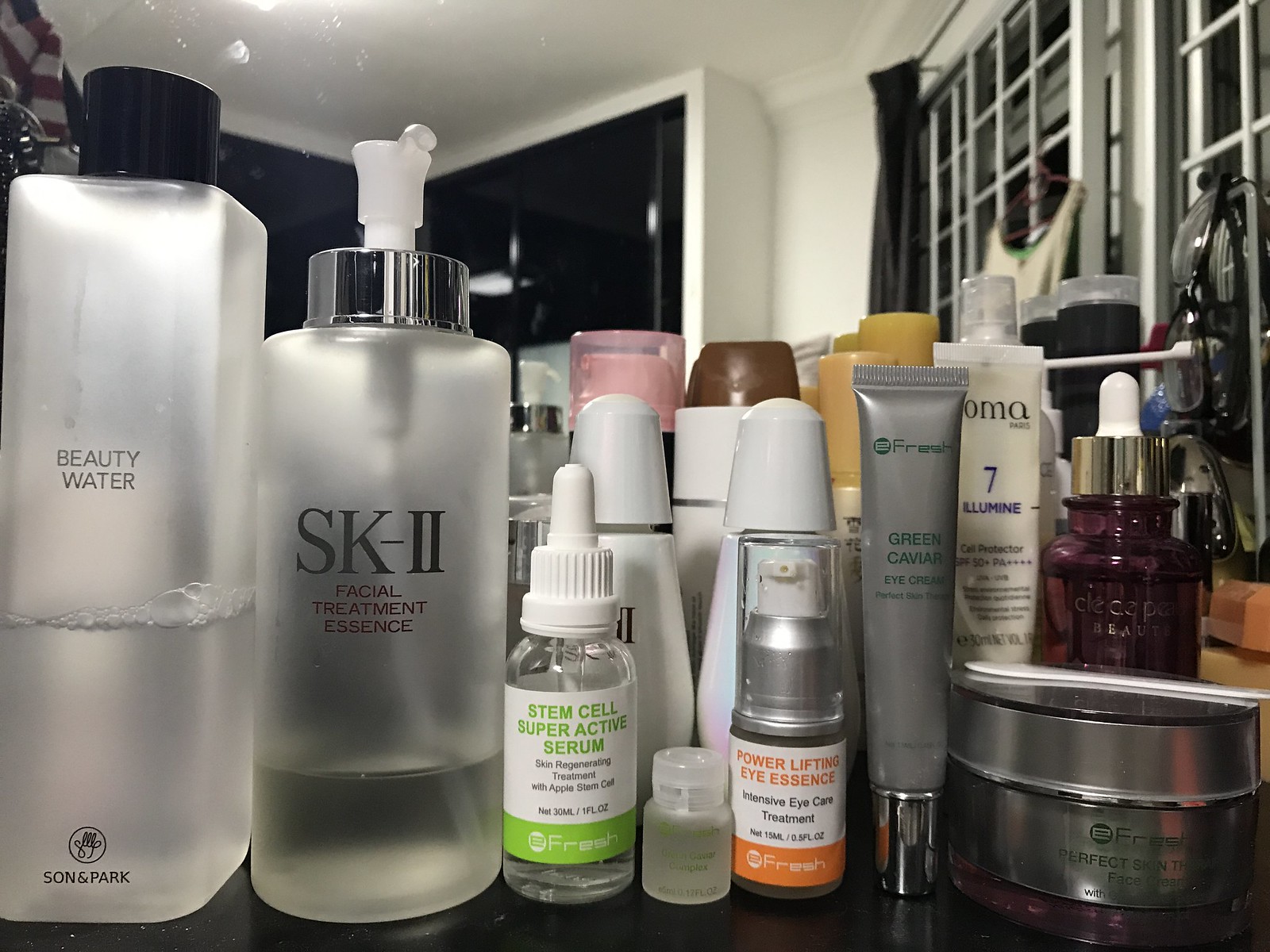This detailed photograph captures a close-up view of an array of skincare products meticulously arranged on a sleek black countertop in a kitchen. The kitchen itself features a contrasting design with white shelving that reveals a stark black interior, framed by white cabinetry. This backdrop includes a white ceiling with a noticeable reflection from an overhead light, enhancing the brightness of the room. On the right side of the image, black curtains are partially open, revealing a window composed of numerous small panes segmented by white cross-hatching.

The countertop hosts an assortment of skincare products, each distinct in its own packaging and branding. Starting from the left, the largest bottle prominently displays "Beauty Water" in a clear glass bottle with a black cap. It is labeled with "Sun and Park" and a logo near the bottom, and appears to be only a third to half full. Next is an SK-II Facial Treatment Essence bottle, recognizable by its silver metallic top and clear liquid content, which is approximately a quarter full.

Following this, a smaller bottle labeled "Stem Cell Super Active Serum" advertises its skin regenerating treatment with apple stem cells. This product bears a green label at the bottom with the brand "Fresh" and holds 30 milliliters or one fluid ounce of content. Behind it stands a white bottle and another with a pink cap, though their labels are obscured.

Adjacent to these, a minuscule bottle sits next to a larger one labeled "Power Lifting Eye Essence," which offers intensive eye care treatment in a net 15 milliliter, or 0.5 fluid ounce capacity. This product features an orange label at the bottom, with "Fresh" branding and orange lettering near the top.

Further along, a cream-like bottle marked with "E-Fresh" and "Green Caviar Eye Cream" is partly visible, as some text remains unreadable. An adjacent bottle shows "OMA Paris" with most of the initial brand name obscured. This product details "7 Ellume" and "Cell Protector," implying its protective skin care function.

Additional bottles fill the remaining space; one notable container has a purplish hue and faintly readable text ending with "CLEAEP Beauty." The collection concludes with a silver tin labeled "E-Fresh Perfect Skin Face Cream," albeit with an incomplete description.

Together, these skincare products create a visually rich and diverse collection, artfully displayed against the sophisticated kitchen setting.